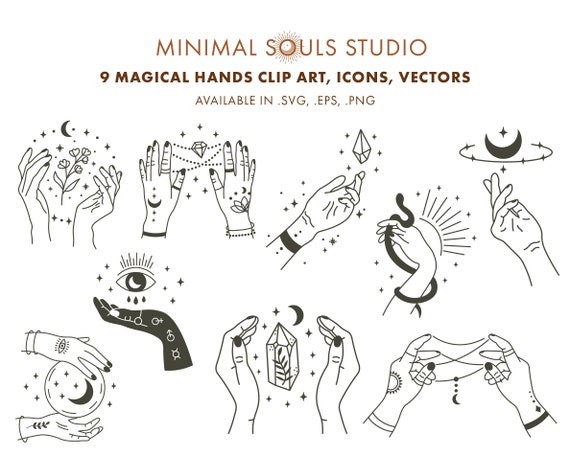The image is a detailed, colorful advertisement for Minimal Souls Studio, showcasing their "Magical Hands Clipart, Icons, and Vectors" available in .svg, .eps, and .png formats. At the top, the text "Minimal Souls Studios" appears, with the "O" in "souls" stylized as a moon silhouette with transparent lines extending outward. Below this is the text "9 Magical Hands Clipart Icons and Vectors."

The background of the image predominantly features black and white illustrations with brown and burgundy tones in the text. The artwork consists of nine detailed images of hands, mostly depicted as feminine, each performing various magical tricks and adorned with distinct tattoos and accessories, such as moons, stars, flowers, and jewelry.

One set of hands is cupped, holding a glowing orb containing a crescent moon and stars, with an eye tattoo and bracelets on the wrists. Another pair holds a plant-studded jewel, evoking a sense of growth and mysticism. A single hand showcases a floating diamond with decorative dots and bands. One striking image features a hand wrapped in a snake, surrounded by celestial symbols. Another has a dark hand marked with sex symbols, an eye, and dripping teardrops, exuding an enigmatic aura. There are additional pieces where hands hold beads, flowers, and strings with pendants, all intricately detailed with moon, sun, and plant motifs.

Overall, this advertisement meticulously presents the studio's intricate and whimsical hand-themed vector art, emphasizing their detailed and mystical style.